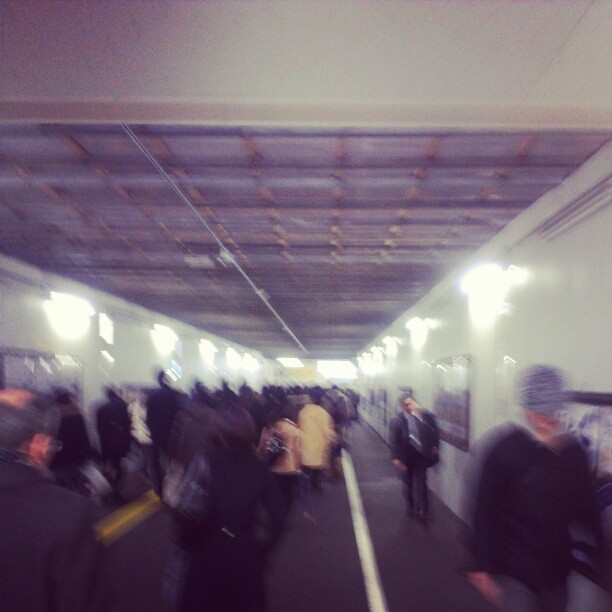A blurred and busy scene captures the hustle of pedestrians navigating a transit hub, possibly an airport, train station, or subway platform. The dark floor features distinct stripes, directing the flow of people moving hurriedly in opposite directions. Wall graphics and evenly spaced light fixtures provide visual interest, while the ceiling showcases a complex plaid pattern, reminiscent of electrical conduits or vents. The crowd, dressed in a variety of attire from casual coats to formal sport coats and ties, adds to the bustling atmosphere. Among them, a man is seen carrying a case, likely containing a suit or sport coat, emphasizing the commuting or travel context of the image.